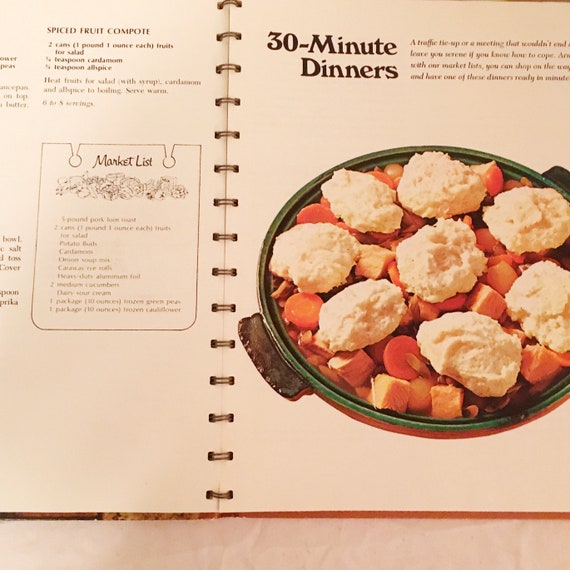The image depicts two open pages of a spiral-bound cookbook. The right page features a section titled "30-Minute Dinners," with a photograph of a pot or bowl containing an off-white dish that appears to be dumplings or biscuits. These are surrounded by chopped carrots and potatoes, suggesting a stew or hearty meal. The left page displays the partial recipe for "Spiced Fruit Compote," while a small, hard-to-read section labeled "Market List" is visible beneath it. The cookbook's pages have a vanilla-like appearance, with small, intricate fonts, and the book's wire binding adds a practical touch.